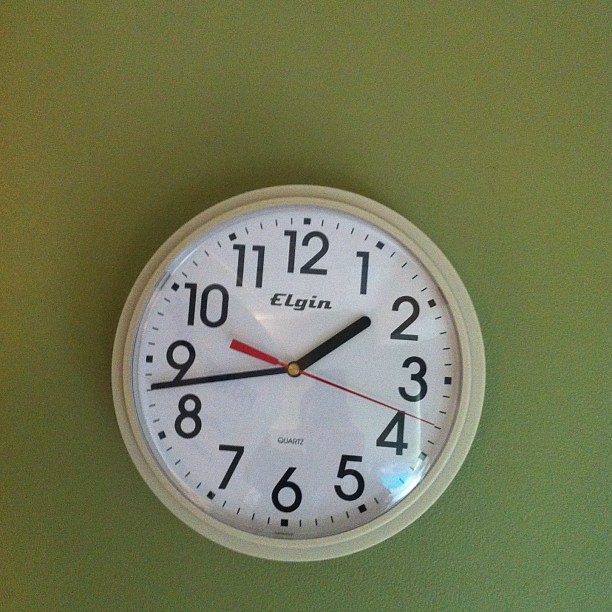This high-quality photograph captures a circular wall clock mounted on a sage green wall, highlighting the subtle nubbing texture of the paint. The clock's body is a slightly off-white hue, while the clock face is a crisp snow white. The brand name "ELGIN" is prominently displayed at the top of the face, with the word "Quartz" in black font positioned just above the number six. The clock features black numbers and dash marks indicating minutes. It has two black clock hands for the hour and minute, and a vibrant red second hand, all three mounted at the center by a small gold circle. A soft light reflection is visible on the clock face, subtly revealing some indistinct shapes.